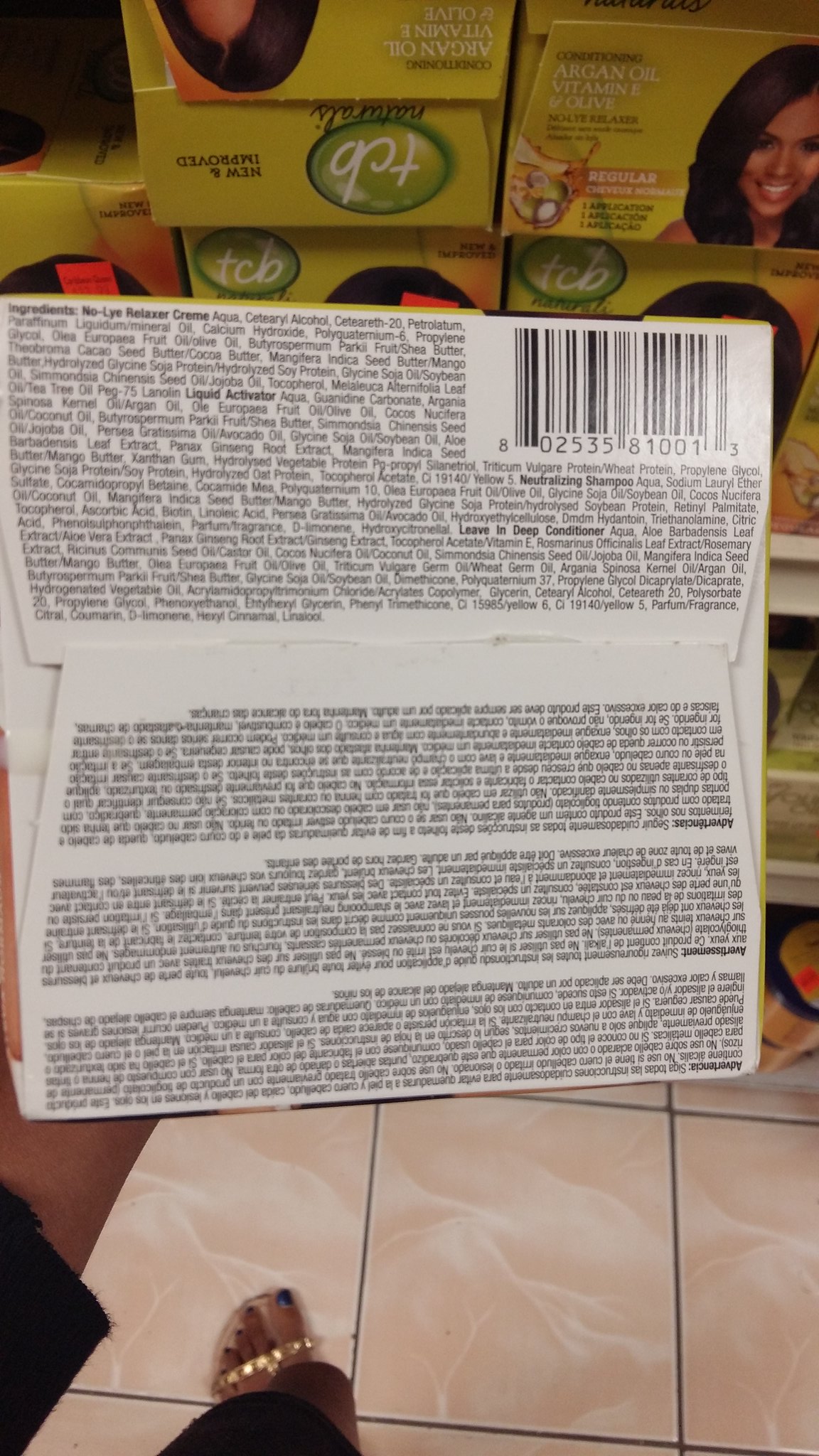This photograph features a detailed close-up of a woman holding the back of a white box with her left hand. The box displays its ingredients prominently at the top, accompanied by a very large barcode in the top right corner. Below, the same ingredients are listed in different languages including English, Spanish, and likely French, but the text is so small and upside down that it's unreadable from this angle. The box appears to be flattened to allow better visibility of the tiny black letters. 

In the foreground, her left foot is shown adorned in a strappy sandal with a striking gold strap. Her toenails are painted green, and she has notably long toes. She is wearing a black dress that exposes part of her knee, and part of a black sleeve is visible in the bottom left corner of the image.

The background of the photo reveals a tan tile floor with gray grout. Additionally, there are other colored boxes, notably yellow and green ones featuring a green circle with the text "TCB" and an image of a brown-skinned woman with dark brown hair. These boxes potentially advertise products containing argan oil, vitamin E, and olive oil, hinting at some sort of conditioning hair treatment. Overall, the scene is meticulously detailed, capturing numerous elements and textures within the frame.